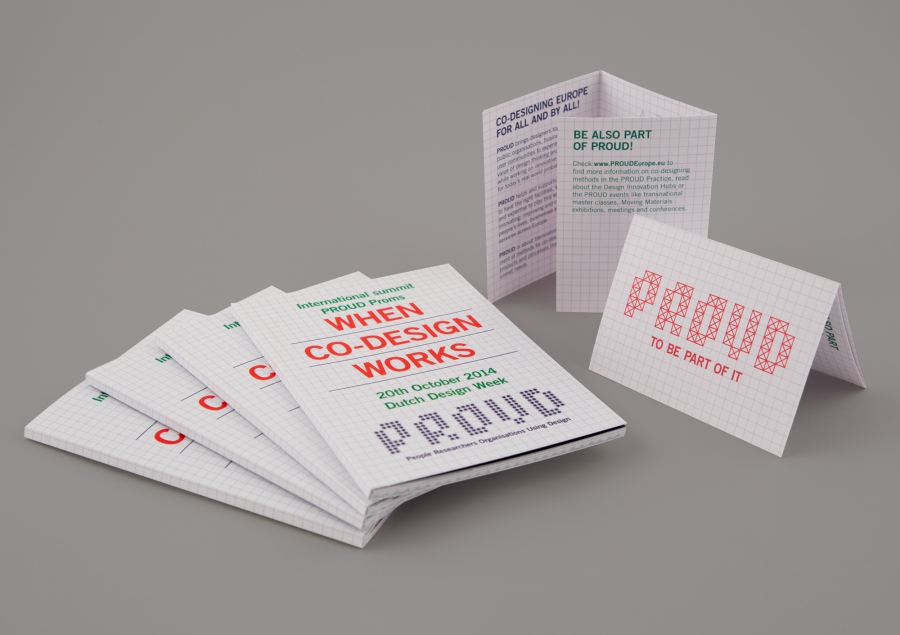The image depicts an array of pamphlets arranged meticulously against a smooth gray background. At the foreground, four pamphlets are laid out in a fan-like structure, anchored at the lower left edge and gently fanning out like the petals of a flower. These pamphlets are titled "International Summit Proud Proms" with the subtitle "When Co-Design Works" in prominent text. Below this are the details "20th October 2014, Dutch Design Week," and a stylized dotted text spelling "Proud." 

To the right of these, there is a trifold flyer standing upright with a blue and green text that reads "Proud to be part of it." Adjacent to this, a horizontally laid-out flyer resembles a postcard, emblazoned with the word "Proud" in red letters, and features the phrase "Co-Designing Europe for all and by all, be also part of Proud." The background’s neutral gray tone enhances the vibrant colors and meticulous design of the pamphlets, generating a cohesive and striking visual presentation of the materials from the summit.